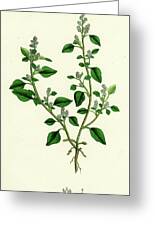The image depicts a plain white greeting card, featuring a delicate and intricately detailed illustration at its center. The drawing portrays a small, forked plant branch with slender, teardrop-shaped leaves in varying shades of green. Vertical, possibly purplish or white flowers bloom modestly among the foliage. The roots of the plant are visible at the bottom of the stem. Encircling the card is a dark gray border, adding to the minimalist and elegant design. At the bottom of the card, there is small, indistinguishable, possibly gray or black writing. The card is devoid of any other text, both on the inside and outside, and displays a subtle, textured background, reminiscent of Victorian-style artistry.